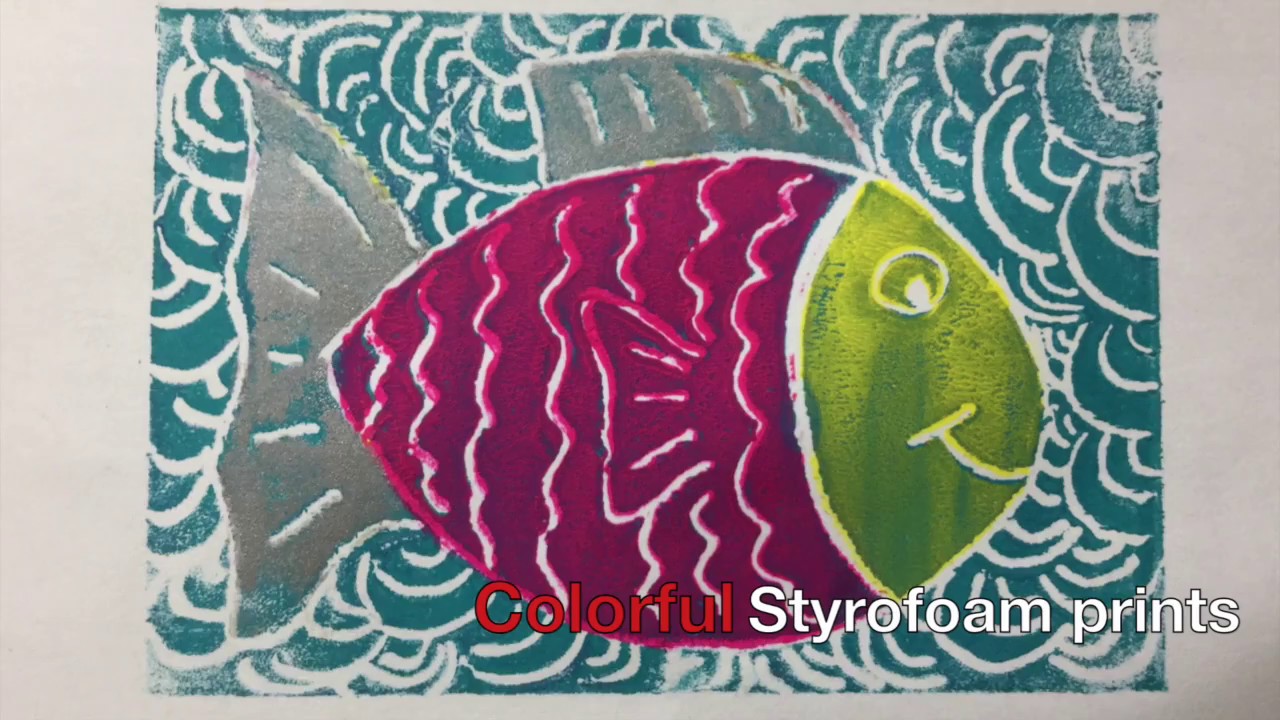This is a vibrant image of a fish depicted through a colorful styrofoam print. The fish, likely a goldfish, exhibits a fuchsia-colored body contrasted by a lime green face, with silver fins adorning its top, back, and tail. It is positioned sideways, showcasing one eye and a cheerful smile. The background features dark blue circular wave patterns against a white backdrop. The bottom right corner of the image contains the label "colorful styrofoam prints," with the word "colorful" in red font and "styrofoam prints" in white. The artwork is created on an approximately eight by eleven-inch piece of paper, placed on a white surface, possibly a table or wall, illuminated by light from above.